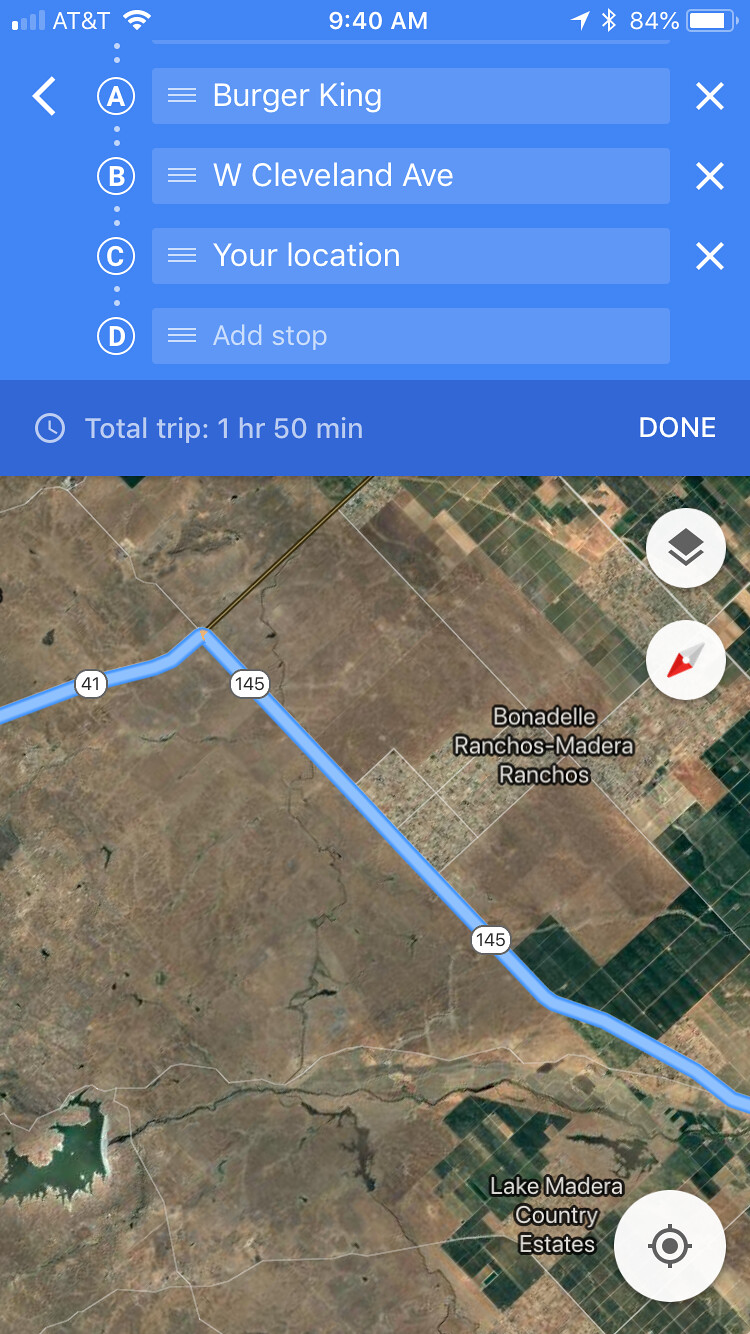This is a detailed screenshot from a mobile phone's map application, specifically showing an aerial satellite view of an urban area. The prominent blue route, marked as 145, stretches from the bottom right of the image towards the left, with a branch labeled 41 veering off to the left. The map predominantly features brown and green squared areas indicating varied topography, with a smaller body of water situated in the lower-left corner.

Key locations on the map include "Bonadel Ranchos, Madera Ranchos" and "Lake Madera Country Estates," both marked in white text. At the top of the image, a blue banner provides navigational details: "Burger King, West Cleveland Avenue, your location, add stop," and states the total trip duration as "1 hour 50 minutes." This blue banner is adorned with white text and includes interactive elements next to each label. There is additional information at the very top of the screen such as the time (9:40 AM), Wi-Fi signal strength (AT&T), and battery status (84%).

The map is visually detailed, blending satellite imagery with highlighted routes and notable identifiers, encapsulating various navigational and location-specific details all within one interface.